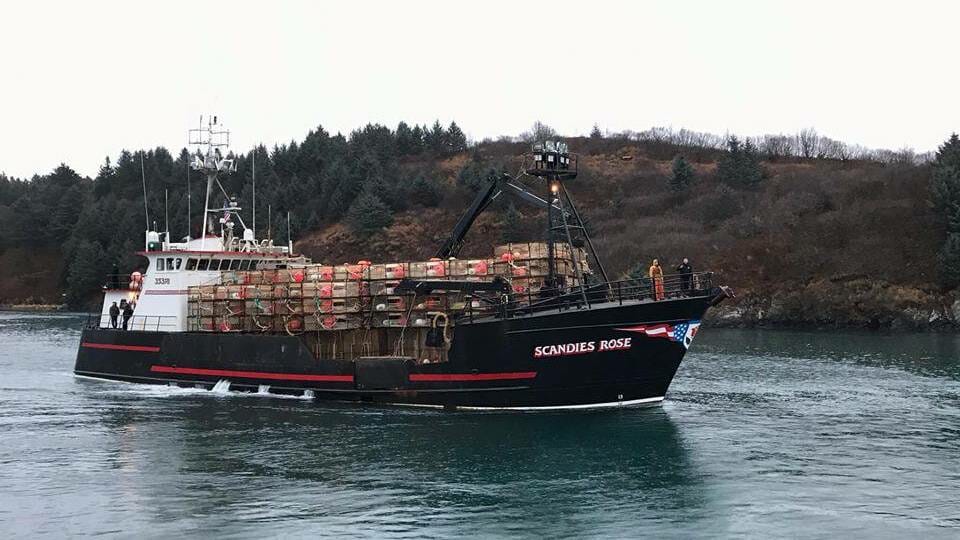This is a horizontal photograph of a large fishing vessel named *Scandies Rose* sailing in the water, likely entering a harbor. The ship's hull is predominantly black with red and white stripes at the waterline and a red, white, and blue decal at the prow. The vessel's name, *Scandies Rose*, is prominently displayed in white letters on the bow. The ship's deck is stacked with crates, possibly containing fish or other cargo, and a black crane is visible in the background. The white-painted wheelhouse, or bridge, is located at the stern, where two men are leaning on a metal railing. Additional crew members can be seen at the bow, overlooking the railing. In the backdrop, there is a brown hill peppered with pine and bare trees, against a white sky. The water beneath the ship appears green, and a gentle white wake suggests the ship is moving at a slow speed.